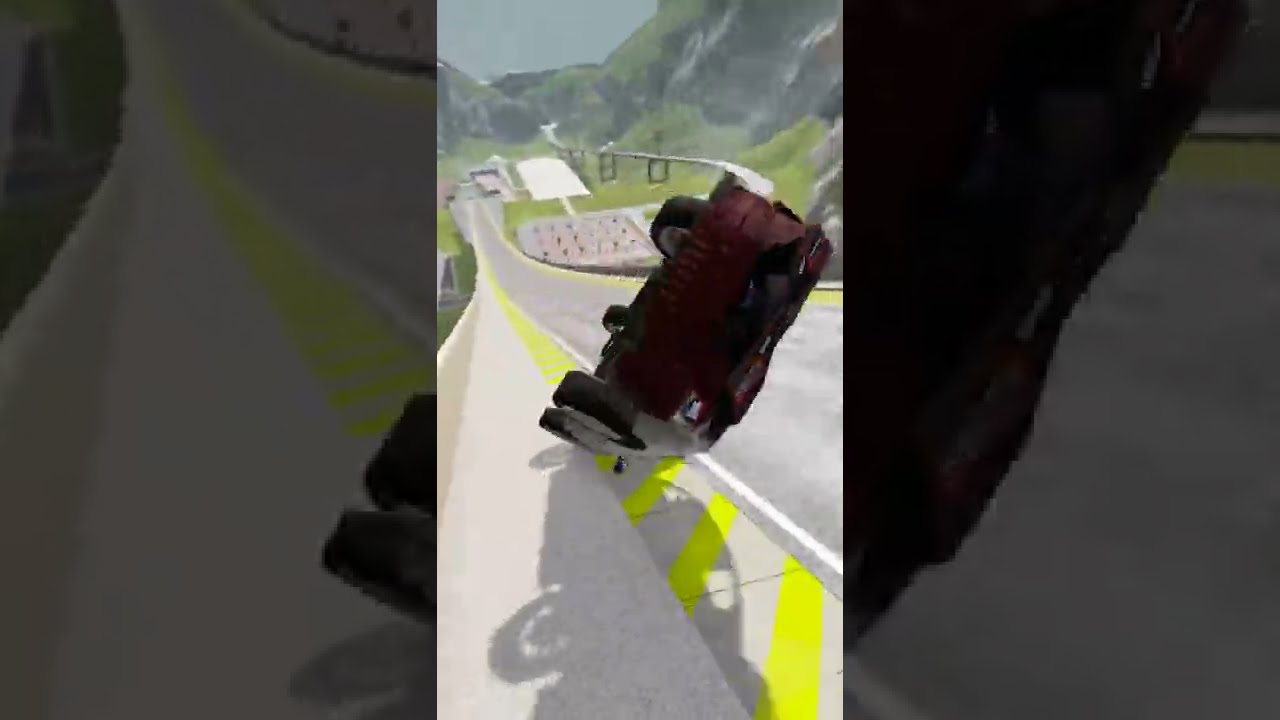The image, captured from a video game, prominently features a red race car in the midst of flipping over on an extremely steep, downhill asphalt roadway. The car, visible in a narrow central strip of a horizontal rectangular image, showcases all four tires and silver rims, with the scene enhanced by an up-close, background view on both vertical sides of the main strip. The road, marked with yellow diagonal caution lines and a central white stripe, runs from right to left and is bordered by a concrete barrier. The steep roadway transitions into a track that curves and swerves down through large, rocky hills. In the distance, the landscape reveals steep mountains with exposed cliff faces and a lush valley, complemented by a bridge and a parking lot. There's water visible beyond the mountains, under a sunlit sky. The close-up side images highlight different parts of the red and gray car, with details of the wheels and end of the car, against the background of the road and surrounding scenery.